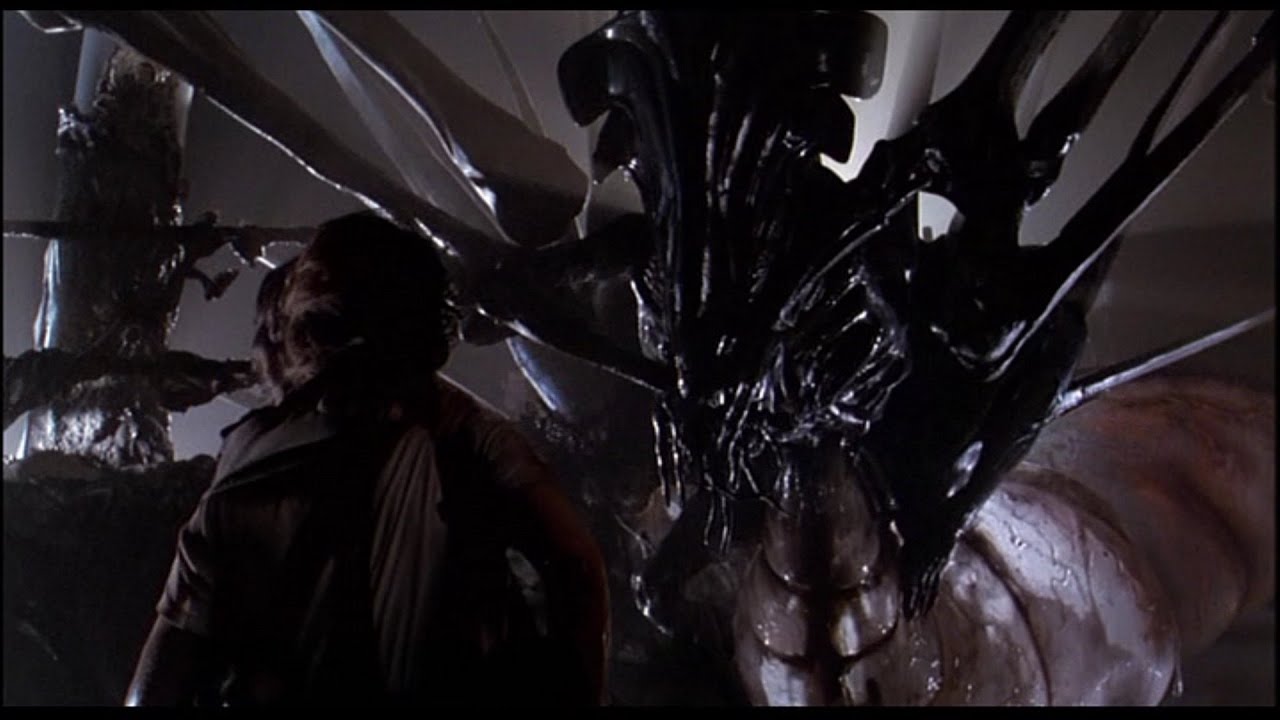This dimly lit photograph, possibly a screenshot from the film *Aliens*, captures a menacing and shadowy scene. Dominating the center of the image is the towering figure of the alien queen, recognizable by her larger and more intricate physique, with pointy, translucent sections flanking her sides. She appears to rise from a cocoon-like, worm-shaped structure that extends downward and behind her, further amplified by her alien head with features resembling medieval weapons protruding from it. A faint light streams in from behind, contrasting with the dark, almost black surroundings. To the left of the alien queen, there is a figure shrouded in shadows, likely Sigourney Weaver's character, standing before the imposing creature. The scene exudes a chilling and sinister atmosphere, emphasizing the sense of looming danger and tension.